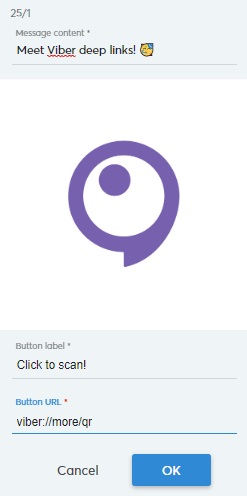The image depicts a slightly blurred printout featuring a range of visual and textual elements. At the top of the printout, the text "25 over 1" is visible, followed by the phrase "message content meet Viber deep links" alongside a logo that incorporates blue and yellow colors. Dominating the central part of the printout, a large purple logo stands out against a white background.

Below this logo, a row of interactive elements is shown, spanning from left to right: a button labeled "click to scan," and a URL highlighted in blue ("Viber: //more/QR") with a red dot positioned just underneath it. Beneath this row, the word "cancel" is present on the left side, while a blue box containing the word "ok" in white print is located on the right.

The design and text suggest that this printout might be a page from a programming or development interface, likely intended for internal use rather than for the public. Throughout the visual, the text appears on a gray background, except for the large purple logo which is set against a white background.